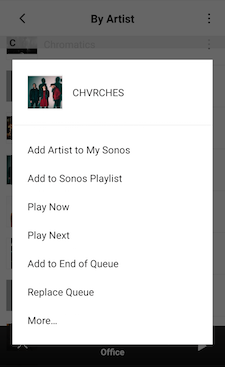A screenshot captures the interface of a music app, presumably Sonos, on a smartphone. At the top, there is a back arrow labeled "By Artist," currently displaying the letter "C," but this entire section appears grayed out. Dominating the screen is a white pop-up featuring the name "CHVRCHES" spelled out with stylistic capitalization (C-H-V-R-C-H-E-S), and it appears to be showcasing an album cover displaying a group of people with their shadows casting on a background wall.

Below the pop-up, several menu options are visible:
- Add Artist to my Sonos
- Add to Sonos Playlist
- Play Now
- Play Next
- Add to End of Queue
- Replace Queue
- More

These options suggest various ways to interact with the artist's music within the Sonos app. A black bar is seen at the bottom of the screen, which is somewhat grayed out but displays the word "Office." To the left, partially obscured by the white pop-up, small thumbnails peek out, hinting at additional content or options.

Interestingly, there are no visible battery meters or typical smartphone status icons, indicating this screenshot might be deliberately cropped to focus solely on the app's interface rather than the entire screen.